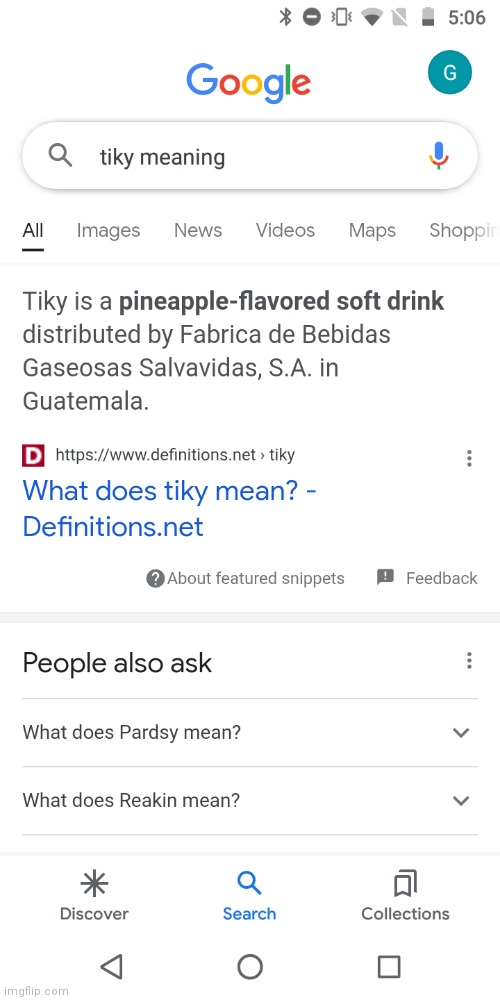This image is a screenshot of a Google search page on a mobile device. At the very top of the page is the familiar Google logo, immediately followed by the search bar. The term entered in the search bar is "Tiki," referring to a pineapple-flavored soft drink. Below the search bar are various tabs for different types of search results: All, Images, News, Videos, Maps, and Shopping. The "All" tab is currently selected. 

The first result displayed is a snippet from definitions.net, providing a brief description of "Tiki." It explains that Tiki is a pineapple-flavored soft drink distributed by Fabrica de Bebidas in Guatemala. Below this description, the search results continue with more information related to "Tiki."